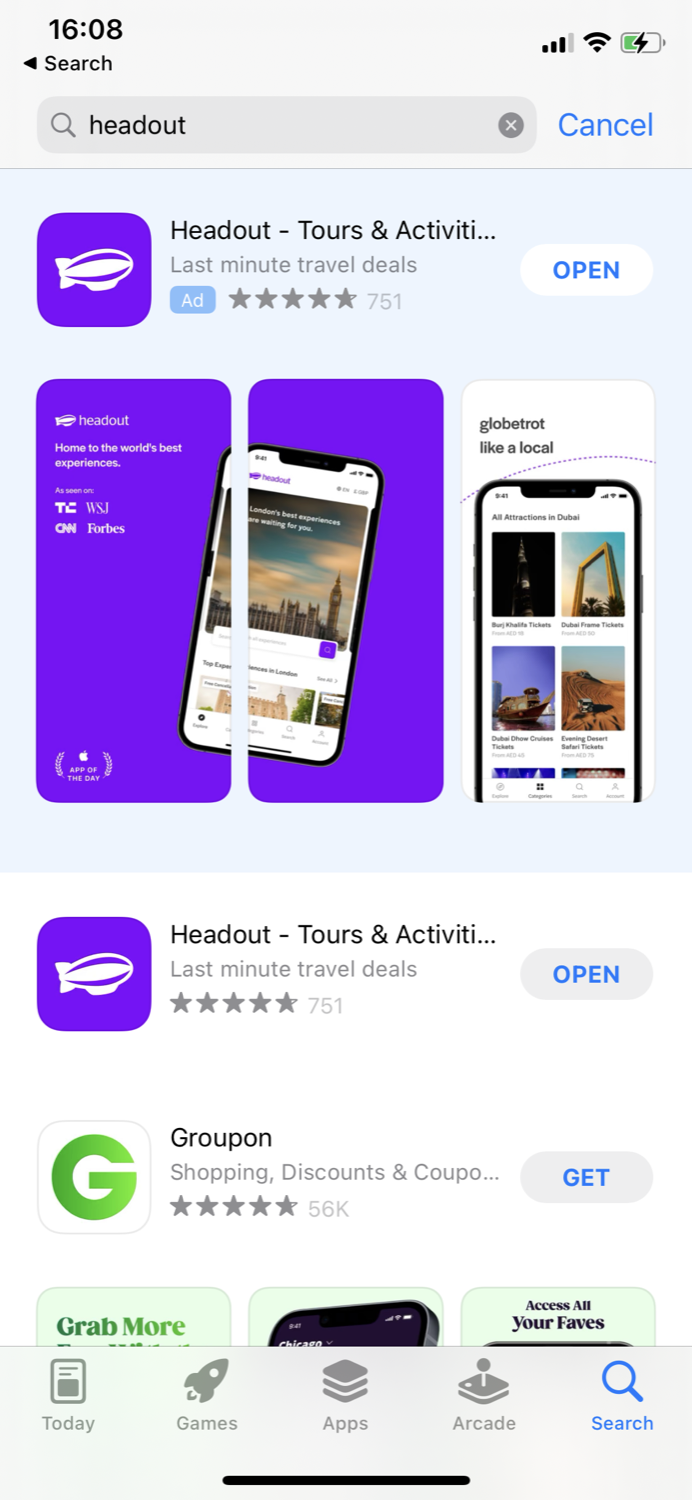The screenshot from a smartphone displays the interface of the App Store. The top border is a light gray, showcasing the standard status icons: the time "16:08" in a 24-hour format on the left, and on the right, the battery icon shows it is half-charged and currently being charged as indicated by a black lightning bolt. Additionally, both the Wi-Fi icon and the wireless signal icon, which highlights four out of five bars for a strong signal, are visible.

The screenshot shows a search result for the term "Head Out" in the App Store. The app in focus is titled "Headout: Tours & Activities," though the text is slightly cut-off. The app's logo features a white blimp within a rounded rectangle. Below the logo, the description reads "Last Minute Travel Deals" and the app boasts a five-star rating, depicted by five gray stars.

Accompanying this are two visual representations of the app interface. The first is a pair of purple vertical rectangles with rounded corners, symbolizing smartphone dimensions. Within these, a small screenshot of the app reveals a stunning panoramic cityscape under a beautiful sky, likely during sunset or sunrise. Adjacent to this, another app screenshot displays four photos including scenic nature shots in the top and bottom right corners. A headline on this screenshot states "Globetrot like a local." 

Located below the "Headout" listing is an advertisement for the same app, showing the same logo and five-star rating. The second listing in the screenshot is for "Groupon," which also has a five-star rating. Groupon's logo is a green letter "G" on a white background.